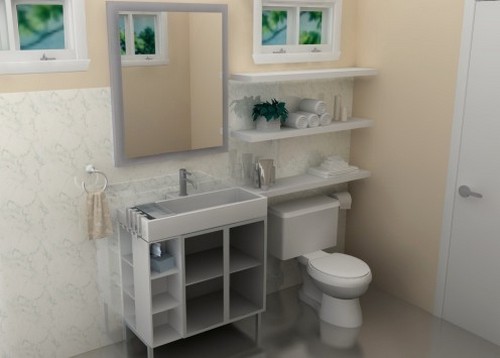The image portrays the interior of a meticulously designed bathroom, which appears to be a 3D model rather than a real-life space. At the center-left, a mirror is mounted above a rectangular sink basin, which is gray in color. Below the sink, there are shelves, with the bottom-left shelf holding a stack of tissues. To the left of the sink, a towel holder is affixed to the wall.

On the top left, a window allows a view of the outdoors, revealing leaves and a portion of the sky. Similarly, at the top right, another window showcases branches, leaves, and more of the sky. In the middle-right section of the room, a toilet is situated, and above it are shelves holding a variety of items, including a potted plant, rolled-up towels, and soaps.

Adjacent to the entrance of the bathroom, the door features a steel frame or door handle, paired with a white door. The walls of the bathroom are painted in a peach hue, contrasting with the back left corner, which has a patterned white grain finish. The floor is composed of brown tiles, adding warmth to the space.

Amidst these descriptive elements, a roll of toilet paper is located in the back right corner of the room. The entire scene, with its precise detailing and lifelike textures, convincingly portrays a 3D-rendered model of a modern, stylish bathroom.